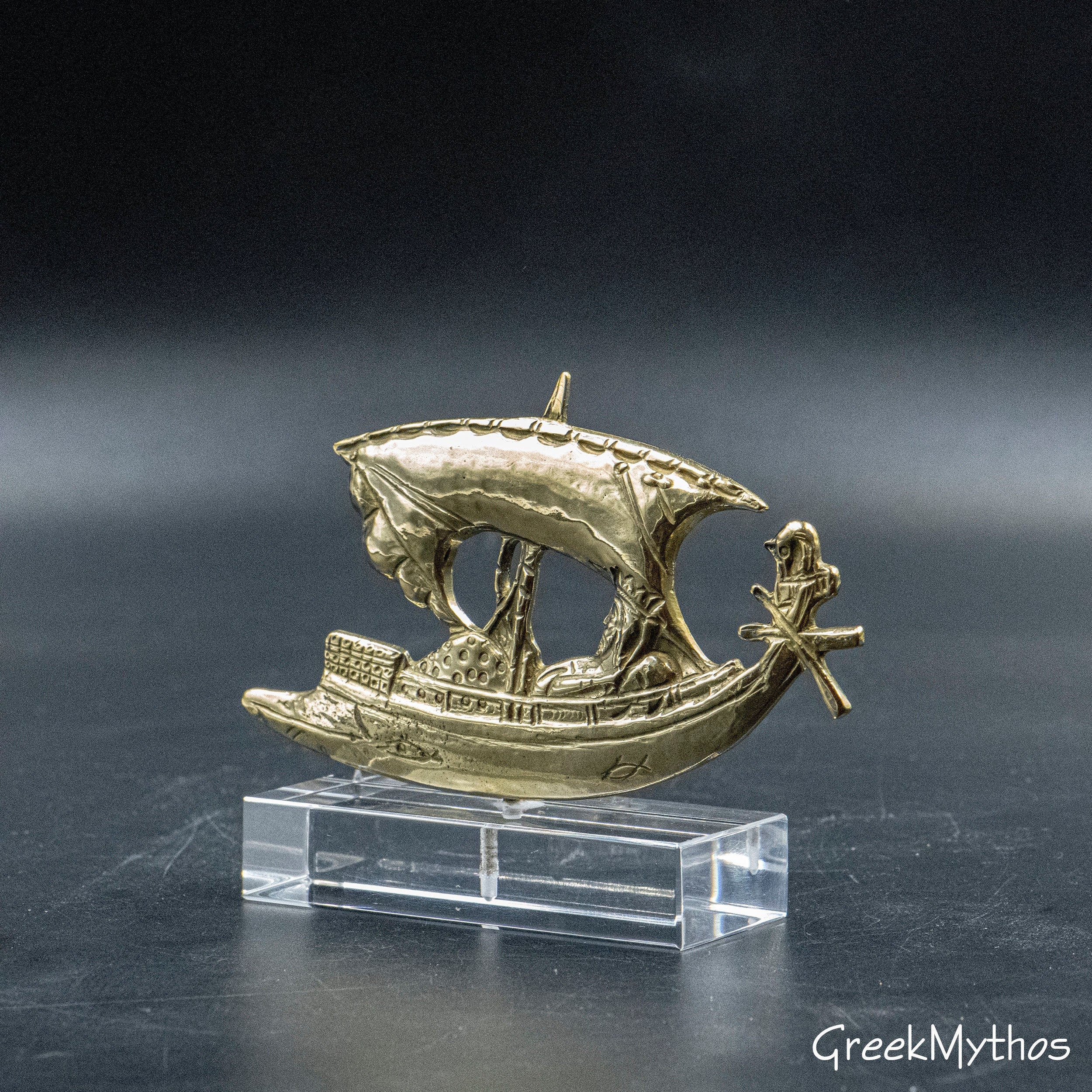The image showcases a miniature Greek ship intricately crafted from gold-colored metal, mounted on a clear rectangular plastic base. The ship is depicted on a dark gray table, which bears visible scratches and dust. The base is only slightly larger than the ship itself, featuring a single peg that holds the ship upright. The ship's design is highly detailed, with artistic carvings that include a fish at the front, intricate patterns, and a railing along the side. The bow of the ship is elevated, with two crossing beams at the top. A sail with a single mast rises above the ship, and a face wearing a crown in profile is visible near the bow. The background transitions from a darkened top to a lighter gray middle, suggestive of a stormy sky or sea. The words "Greek Mythos" are displayed in the bottom right corner in white letters.